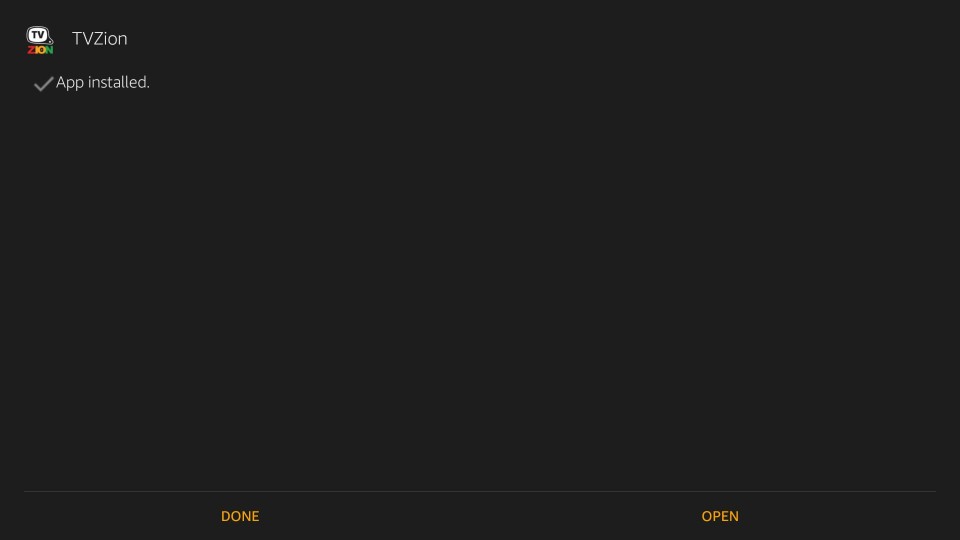Here is the cleaned-up and detailed descriptive caption:

---

This is a large, rectangular, and horizontally oriented screenshot predominantly in dark gray, almost black. The focal point of the screenshot is the installation confirmation for an app called TVZION. In the top left corner, the TVZION logo is prominently displayed. The logo features a small TV icon in white, with the letters "TV" in black inside the TV symbol. Directly beneath the TV icon, the word "ZION" is written with a distinctive color scheme: the letter 'Z' is red, 'I' is orange, 'O' is yellow, and 'N' is green. Next to the logo, the app name "TVZION" is written, with "TV" in uppercase and "zion" in lowercase letters, all in white text. Below this, the text "APP INSTALLED" appears, preceded by a white checkmark, indicating that the installation process has been completed. At the bottom of the screen, there are two buttons: "DONE" on the left and "OPEN" on the right. Both buttons feature orange text.